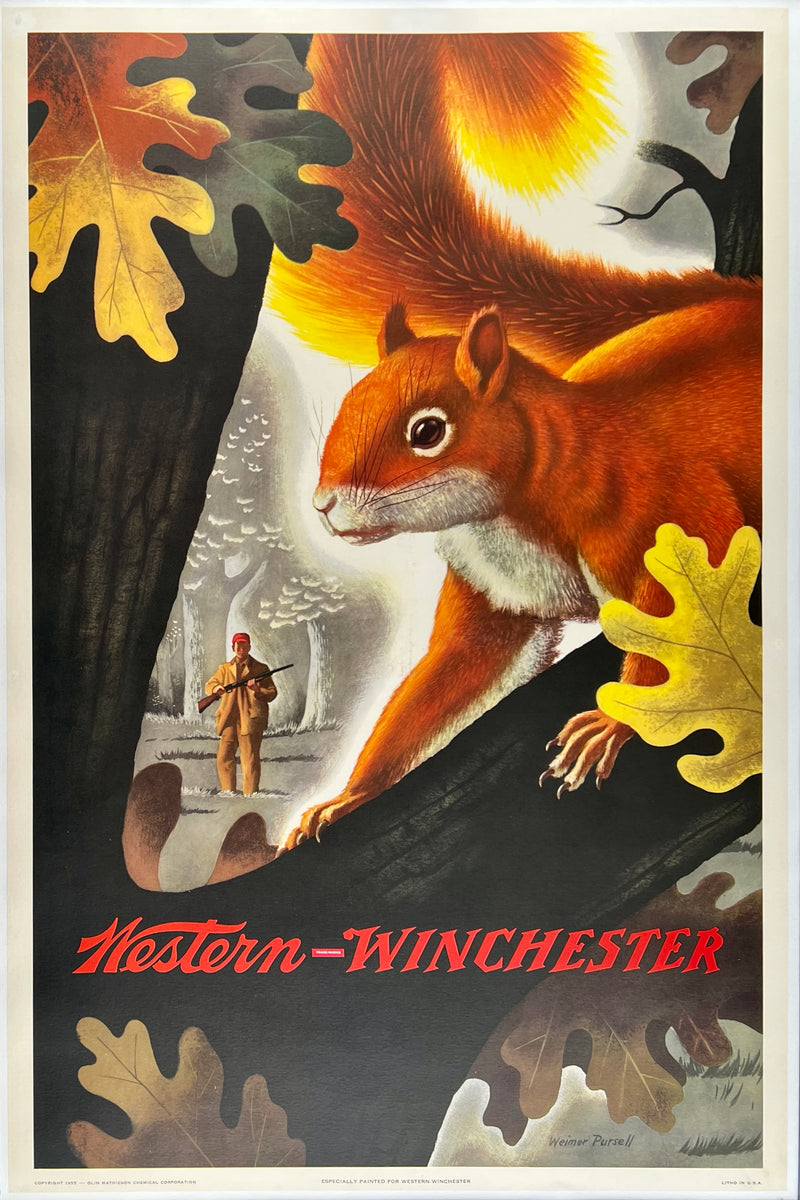The poster is an animated advertisement for a gun, specifically a Western Winchester rifle. The image features a close-up of a tree with large branches, dressed in vibrant fall colors with leaves falling. A big red squirrel with a yellow and brown tail clings to one of the branches. In the background is a man in hunting gear, comprising of all-brown clothes and an orange hat, carrying a rifle. The scene appears to depict him on a hunting expedition, likely for squirrels. The background is predominantly black and white, featuring white trees, creating a contrast that suggests either snow or grass. The text "Western Winchester" is prominently displayed across the bottom of the poster. Shadows and the dark background amplify the focus on the hunter and the squirrel, accentuating the hunting theme of the advertisement.